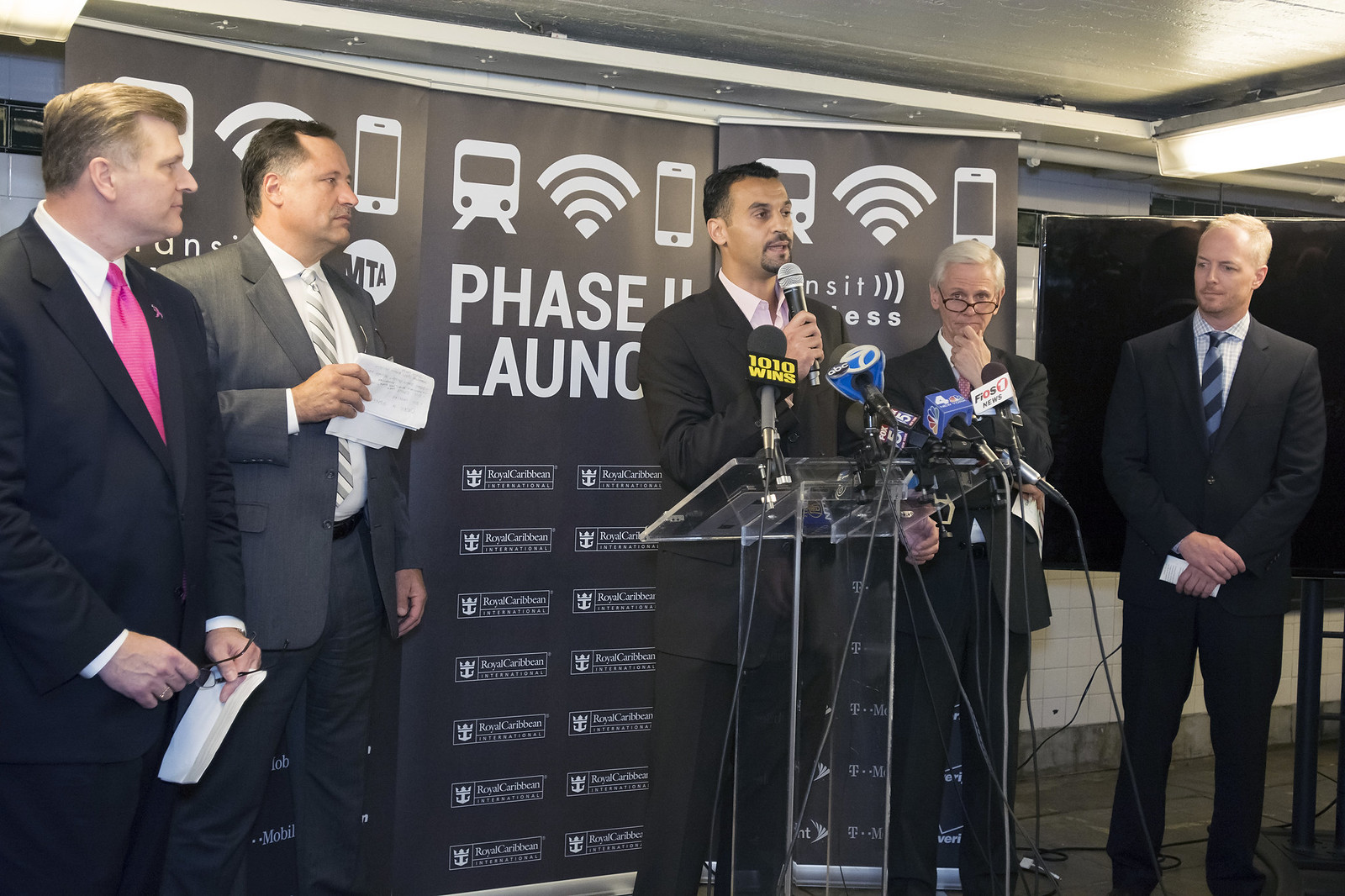The image captures a scene from a well-lit indoor conference, likely an expo, featuring five middle-aged to older white men standing on a stage, all dressed in suits. The age range of the men appears to span from their 40s to 60s. The central figure, a man with dark features, is speaking into a microphone held in his right hand. He stands behind a clear podium, surrounded by multiple microphones. Four other men flank him, two on his left and two on his right, all attentively watching him. They hold folded pieces of paper. 

The men have distinctive attire: the first on the left wears a black suit with a pink tie; the second a gray suit, white shirt, and striped tie; the speaker himself in a black suit with a white shirt; next, a man with white hair, glasses, and a black suit; and finally, a man in a dark brown or black suit with a blue tie. Behind them is a large black poster board displaying the words "Phase 2 Launch" and several icons, including a television, a smartphone, and a Wi-Fi signal. There is a turned-off projector monitor visible to the right, and the ceiling and floor in the background are both a beige color. The overall color palette of the image includes black, white, yellow, gray, silver, and pink.